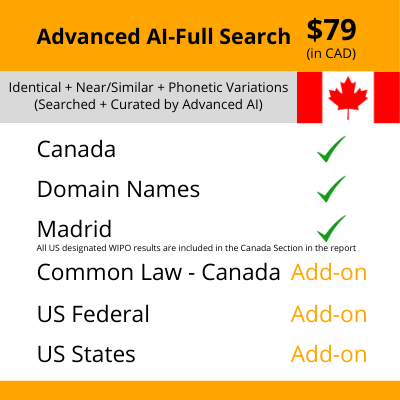The image features a design with orangish-yellow borders at the top and bottom. Within the top border, there's a bold black font text that reads "Advanced AI - Full Search $9.79 (in CAD)," with the "in CAD" portion in non-bold text inside parentheses. Below this, on a gray border, it states "Identical + Near/Similar Phonetic Variations (Search + Curated by Advanced AI)."

The center of the image displays the red and white Canadian flag, featuring a prominent red maple leaf in the middle. The lower part of the image, set against a white background, includes several notable text elements. Firstly, the word "Canada" followed by a green checkmark. Additional text lists the following features with green checkmarks: "Domain Names", "Madrid", "All EU as Designated Repo Results Included in Canadian Section of the Report", "Common Law Canada Add-on", "US Federal Add-on", and "US States Add-on."